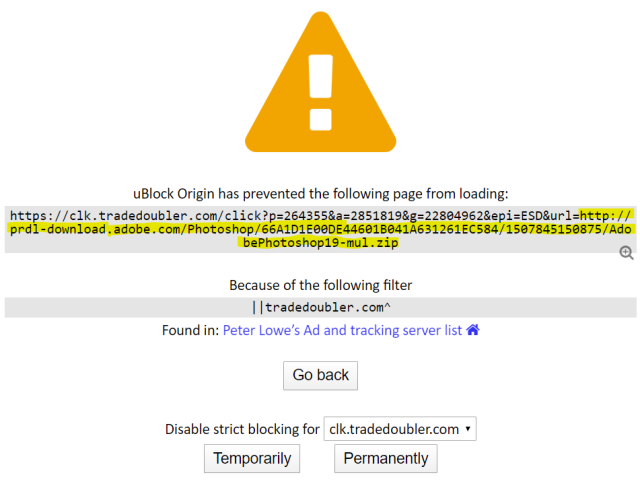**Image Description:**

The image features a warning sign prominently displayed, which is a yellow triangle with a white exclamation mark inside it. Beneath the warning symbol, there is a message stating, "uBlock Origin has prevented the following page from loading:". This message is followed by a highlighted URL, indicating the blocked site: "https://seeok.tradedoubler.com/click?p=264355&a=2851819&g=22804962&EPI=ESD&URL=http://prdl-download.adobe.com/photoshop/66a1d1e00de44601b041a631261ec584/1507845150875/adobe_photoshop_19-mul.zip."

To the right of this URL, there is a magnifying glass icon enclosed in a small gray box, which is typically used to indicate further inspection or detailed view. Below this icon, the text reads, "Because of the following filter:" followed by another gray box containing, "tradedoubler.com ⬆ found in Peter Lowe's Ad and tracking server list." There is a blue hyperlink underneath it, presumably for further information about the filter or the list.

At the bottom of the warning message, there are various interactive elements. There is a "Go Back" button, a "Disable strict blocking for this site" button, and two gray buttons labeled "Temporarily" and "Permanently," suggesting options to either temporarily or permanently disable the blocking for this specific source.